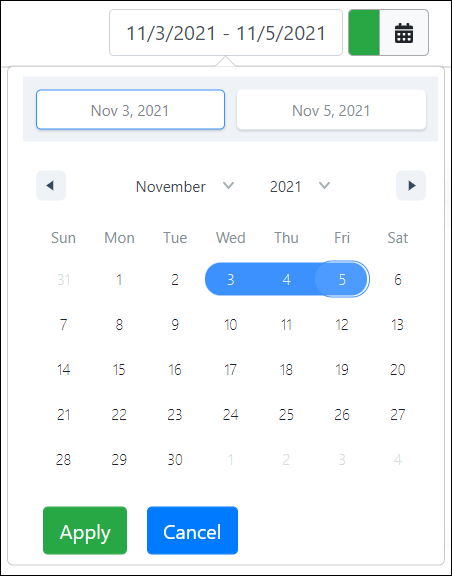A detailed screenshot showcasing a calendar interface is depicted within a white square framed by a black border. At the top of this calendar interface, a rectangle with a thin gray border displays a date range in black text: "11/3/2021 - 11/5/2021," which translates to November 3rd, 2021 through November 5th, 2021. To the right, another small rectangle sports a dark green vertical band on the left and a black silhouette of a calendar on the right.

Beneath this, a light blue rectangular section, bordered by dark green or dark blue, contains two date selectors in gray text. The first reads "NOV 3rd, 2021," while the second, which is not selected, reads "NOV 5th, 2021." 

In the surrounding white area, there is a small square with a dark gray background featuring a left-pointing black arrow. Adjacent to this, "November" and "2021" are displayed with gray drop-down arrows next to each. Another gray square on the right continues the interface elements, containing a right-pointing black arrow.

At the top, days of the week are presented in gray text—abbreviated as SUN, MON, TUE, WED, THU, FRI, and SAT. The days of the month follow: numbers 1 through 30 in black text, while the previous month's 31 and the next month's 1, 2, 3, and 4 are in gray text.  Days 3, 4, and 5 (Wednesday through Friday) are specifically highlighted in blue to indicate the selected date range.

At the bottom, the interface features two rectangular buttons—one dark green with white text labeled "APPLY" on the left and another dark blue with white text labeled "CANCEL" on the right.